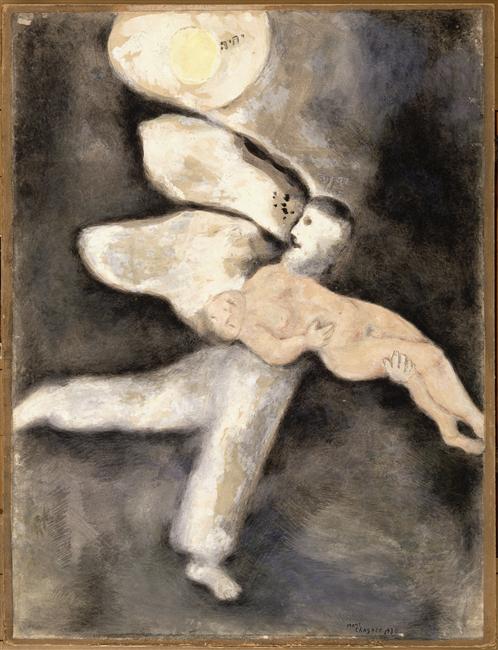In this evocative painting, an abstract scene unfolds against a dark, brooding background of swirling grays and blacks, reminiscent of stormy clouds or ghostly apparitions. At the top of the composition, a somewhat abstract, egg-like moon dominates the night sky with its white outer shell and yellow center, subtly illuminating the scene below. Central to the image, a haunting figure dressed in white—which could be interpreted as an angel or a saint—stands precariously on his left foot, seemingly poised for flight. His expression is one of dismay, with a visible black eye and black hair contrasting sharply with his pallid face. He cradles a nude woman in his arms; her body appears limp and contorted, her eyes closed as if she’s hurt or lifeless. Wisps of white, cloud-like forms emanate from their faces, adding to the composition's ethereal and otherworldly ambiance. This image is framed by a subtle brown outline, grounding the surreal elements within a defined border.